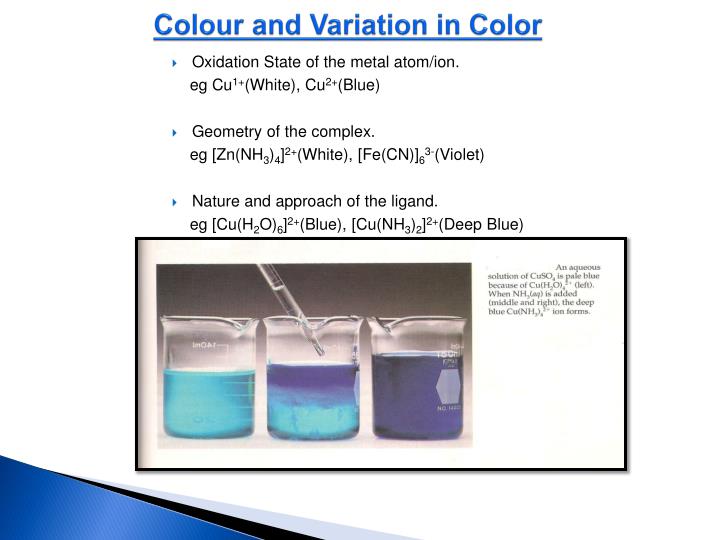The infographic, set against a white background, is titled at the top in bold blue underlined text: "Colour and Variation in Colour," with "colour" spelled in British English initially and American English subsequently. Below the title, there's a section articulated in black text accompanied by three blue arrow-shaped bullet points. The first bullet point states, "Oxidation state of the metal atom/ion," providing examples: Cu^1+ (white) and Cu^2+ (blue). The second bullet point addresses the "Geometry of the complex," with intricate chemical formulas as examples such as Zn(NH3)4^2+ (white) and [Fe(CN)6]^3− (violet). The third and final bullet point discusses the "Nature and approach of the ligand." Below this section, the infographic features a photograph of three beakers containing blue liquids. The left beaker holds a bright blue liquid, the middle beaker shows a light blue liquid being darkened by a dropper from above, and the right beaker contains a dark blue liquid. There is also some additional small text accompanying the photograph, including a reference to an aqueous solution of CuSO4, noting its pale blue color.